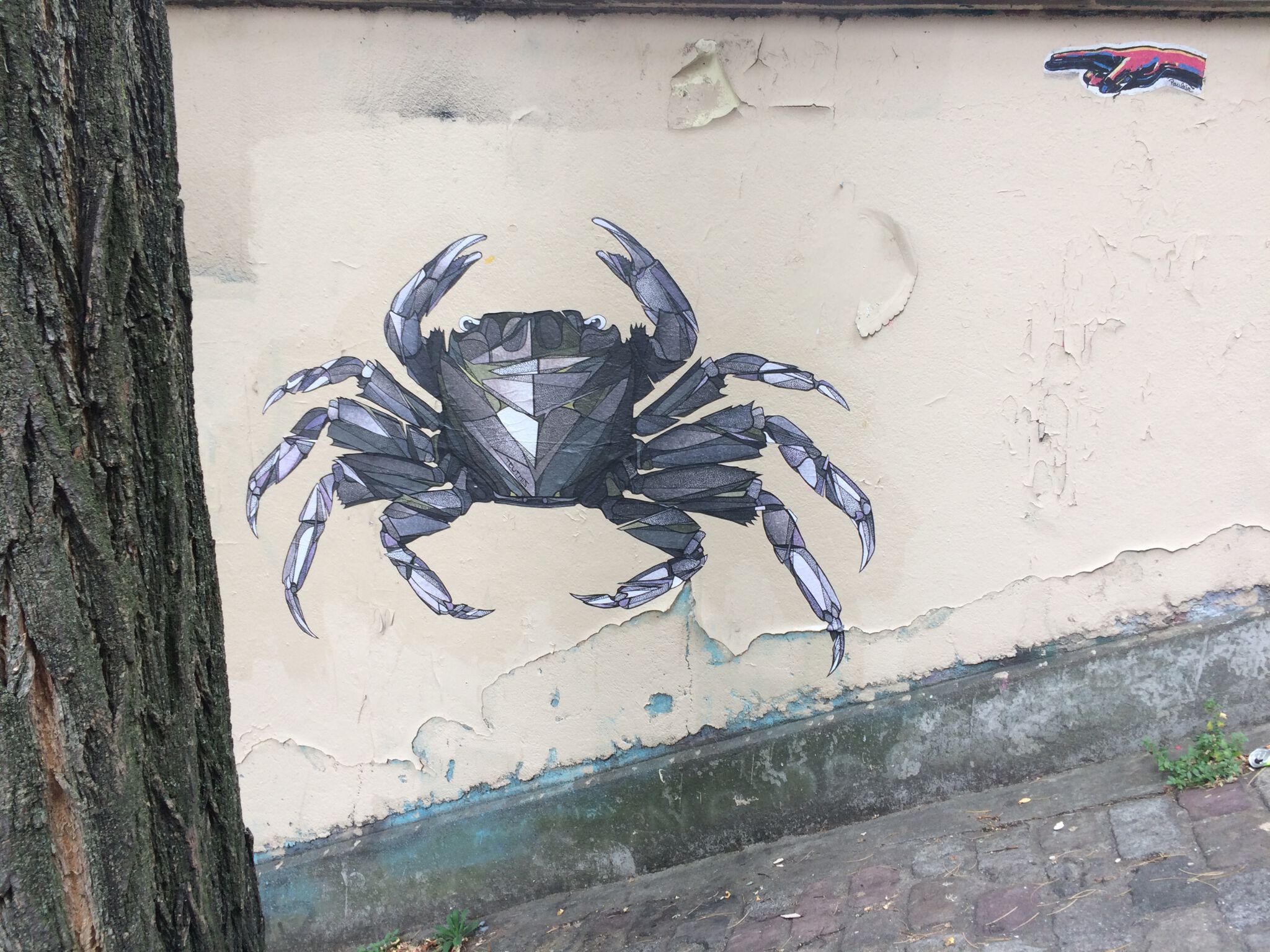The photograph depicts a side wall on a street with a peeling, beige-white paint revealing a teal blue layer beneath, indicating its old and damaged condition. The wall slopes slightly, as if on a hill, and starts at the bottom with cobblestone bricks, red and gray in color. A dark brown tree trunk from top to bottom occupies the left edge. Dominating the wall is a large mural of a crab painted in varying shades of gray and blue, giving it a mosaic-like appearance. The crab’s claws are lighter gray with white accents while its body gradually darkens. In the top right corner of the wall, there's a sticker or small painting of a pink and blue hand making a peace sign.